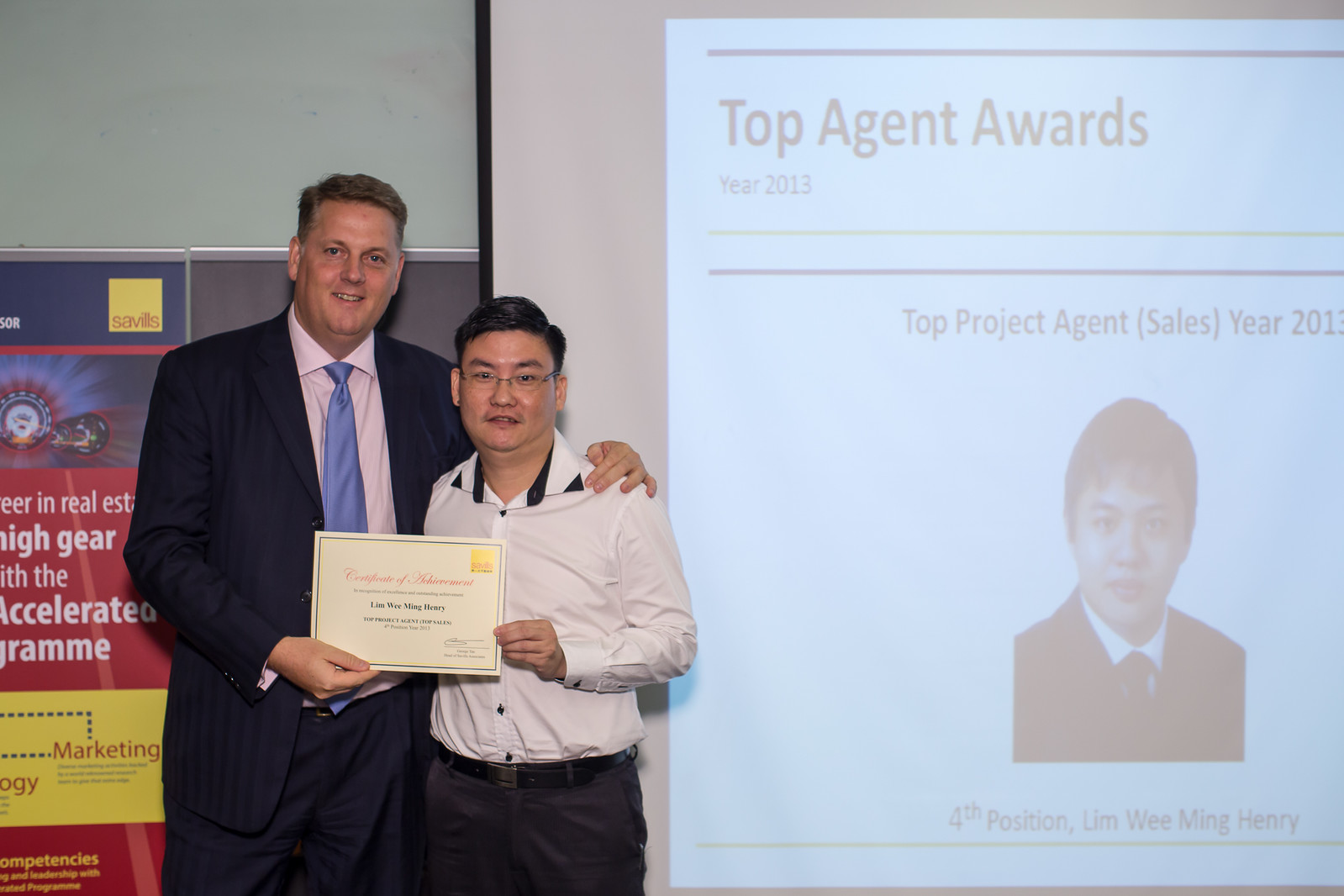In the photograph, on the left side, there are two men posing together with a certificate. The man on the far left is fairly tall, Caucasian with graying black hair, dressed in a navy blue suit, slightly pink dress shirt, and a light blue tie. He has his arm affectionately around the shoulders of the man next to him. The other man, Lim Wee Ming Henry, is of Asian descent, wears glasses, and is dressed in a white long-sleeved button-up shirt paired with black slacks. They are jointly holding a certificate that prominently displays "Certificate of Achievement" in red lettering and includes Lim Wee Ming Henry's name. 

To their right stands a projector screen displaying a PowerPoint slide. The title section at the top, enclosed in two horizontal blue lines, reads "Top Agent Awards Year 2013." Below that, the text says "Top Project Agent (Sales) Year 2013," followed by a photograph of Lim Wee Ming Henry himself. The slide further indicates his achievement by stating "Fourth Position," and repetitively confirms his name, Lim Wee Ming Henry. Towards the left side of the image, there is also a banner featuring the name "Savills," presumably the company associated with the awards and certificate.